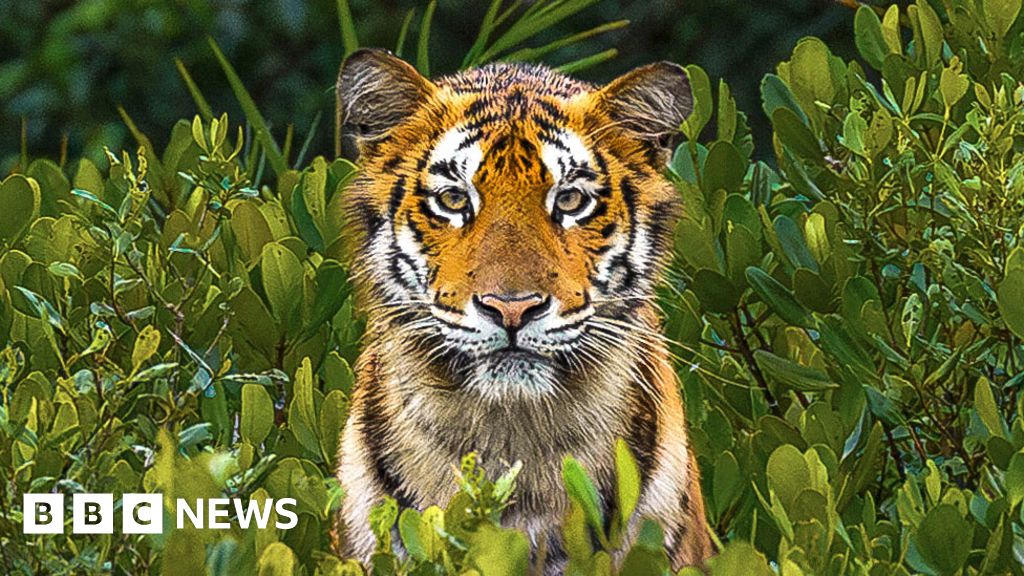In this vivid and detailed image, which appears to be a screenshot from a BBC News video, a young tiger is prominently centered against a lush green backdrop. The tiger gazes directly at the camera with its pale yellowish-green eyes, exuding an air of calm curiosity. Its face is a striking blend of orange with black markings, accompanied by white accents around the eyes, nose, cheeks, and jaw. The tiger's body, visible through partially obscuring leaves, displays its trademark black stripes against a murky coat that transitions between yellow, orange, and white. Surrounded by dense, verdant foliage, the environment suggests a wild habitat rich in tall grass and broad-leaved shrubs. The background is darker and more sparse above the tiger's head, giving depth to the scene. The bottom left corner of the image features a white BBC News logo, giving context to this captivating snapshot of nature.